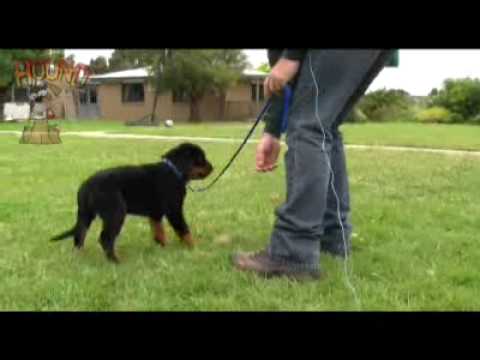In this detailed screenshot from a puppy training video titled "Hound," a man is seen training a young Rottweiler in an outdoor setting. The logo "Hound" is positioned at the top left, arched slightly, with a cartoon-style dog with its tongue sticking out sitting below it. The man, dressed in blue jeans, gray shoes, and possibly a gray sweatshirt, is bending down. His right hand is extended towards the puppy, while his left hand firmly holds the leash attached to the small Rottweiler. The Rottweiler, with its black fur and brown paws, stands at the middle left of the image.

The background features a brown house with a white roof, gray door, and windows, suggesting a residential or possibly a public building. The lawn, composed of short grass, intersects with a diagonal sidewalk leading past the house. Together, these elements create a serene scene for the puppy training session. There's also an indication of recording equipment, seen as a thin wire running down the man's pant leg, emphasizing the professional aspect of this video.